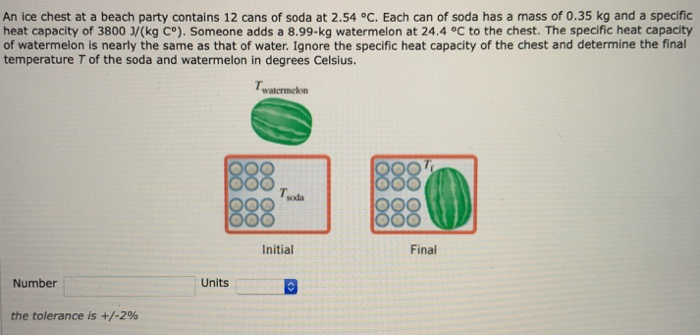The image is an exam question from a textbook that depicts a problem involving thermal equilibrium. At the top of the image, a paragraph states: "An ice chest at a beach party contains 12 cans of soda at 2.54 degrees Celsius. Each can of soda has a mass of 0.35 kilograms and a specific heat capacity of 3,800 J/kg°C. Someone adds an 8.99-kilogram watermelon at 24.4 degrees Celsius to the chest. The specific heat capacity of watermelon is nearly the same as that of water. Ignore the specific heat capacity of the chest and determine the final temperature (T) of the soda and watermelon in degrees Celsius."

The visual section of the image includes a drawing illustrating the scenario: a square representing the chest containing the soda, annotated with "T_soda," and a watermelon labeled "T_watermelon." The illustration shows a transition from an initial state (left) to a final state (right). In the initial state, the items are separate, while in the final state, both the watermelon and soda cans are combined within the chest. 

At the bottom of the image, there is a section for inputting the final temperature in numbers and units, with a tolerance indicated as ±2 degrees Celsius. It specifies that you are to ignore the specific heat capacity of the chest itself. This problem requires calculating the final equilibrium temperature after thermal exchange between the soda and the watermelon.